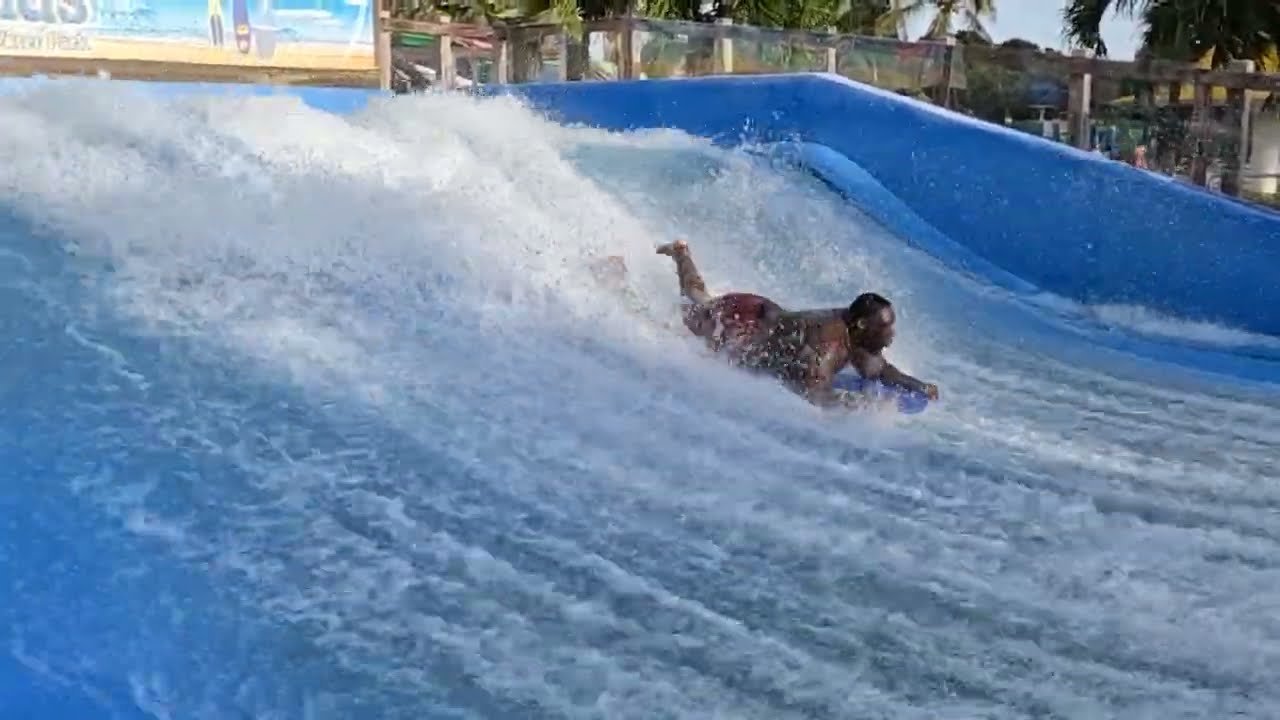The image shows an African-American man with short black hair, riding a purple paddleboard on a large blue artificial wave machine set outdoors. He is shirtless and appears to be wearing red swim trunks, although the water makes it difficult to see clearly. The wave machine generates frothy white water cascading down a hill, creating a dynamic surfing experience. In the background, a brown wood fence encircles the area, with partial views of palm trees and the bottom of a billboard or sign, which seems to depict surfboards and water. Additionally, there is a glimpse of a parking lot with cars, suggesting the location is not on a cruise ship. The man appears to be skillfully managing the man-made wave, possibly participating in a contest given his stable position on the board. The scene is bright and sunny, with some blurry, out-of-focus elements adding to the lively atmosphere.